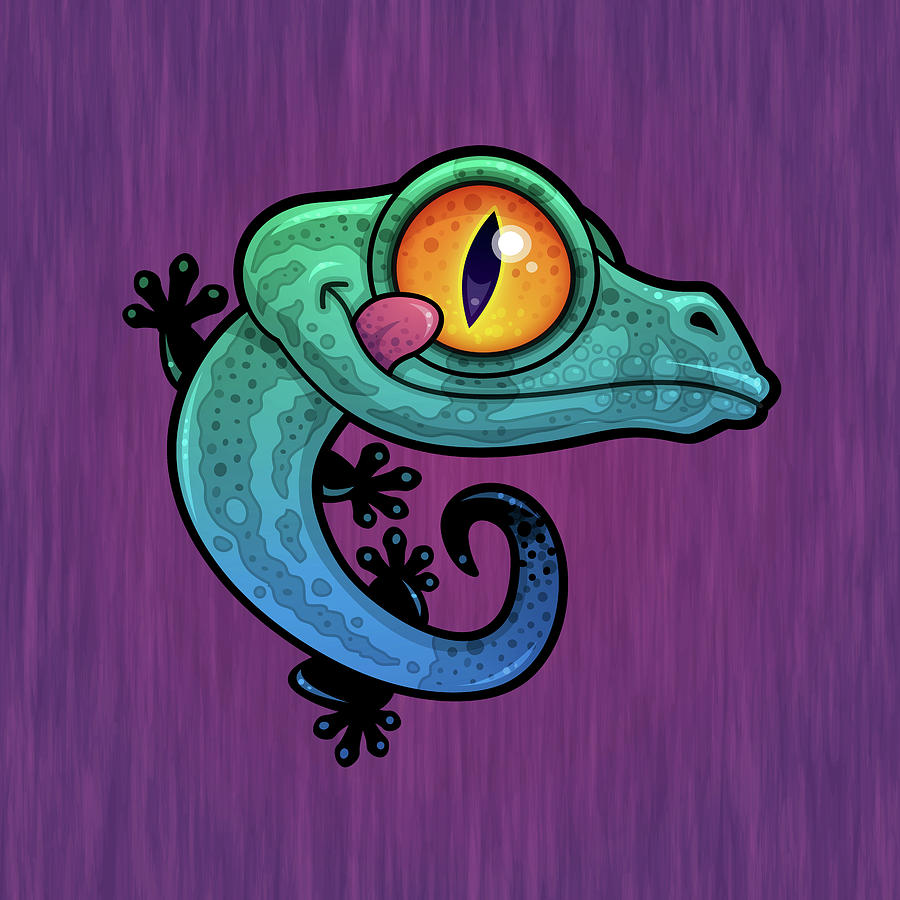In this square-shaped image, approximately six inches by six inches, we see a vividly colorful and cartoon-like chameleon centered prominently. The chameleon, characterized by a disproportionately large head, is crawling up a wall with its body curved towards the right and its tail curled inwards. Its head is turned to the right, showcasing a large, round orange eye with tiny orange dots, a black cat-like pupil edged in yellow, a long nose, and a short snout. Despite its closed mouth, the tongue intriguingly points up towards its eye.

The chameleon's body exhibits a vibrant spectrum of colors with its back in shades of blue, transitioning to green as it moves upward. The legs and toes start as blue and black but shift to green and black closer to the head, creating a dynamic look.

The background consists of vertical swatches in varying shades of purple, which are darker in the four corners and gradually lighten towards the center to a more pinkish hue, artfully enhancing the chameleon’s colorful presence. The overall setting suggests the chameleon as the main character in a whimsical cartoon, brought to life through the artist's use of bold colors and intricate details.